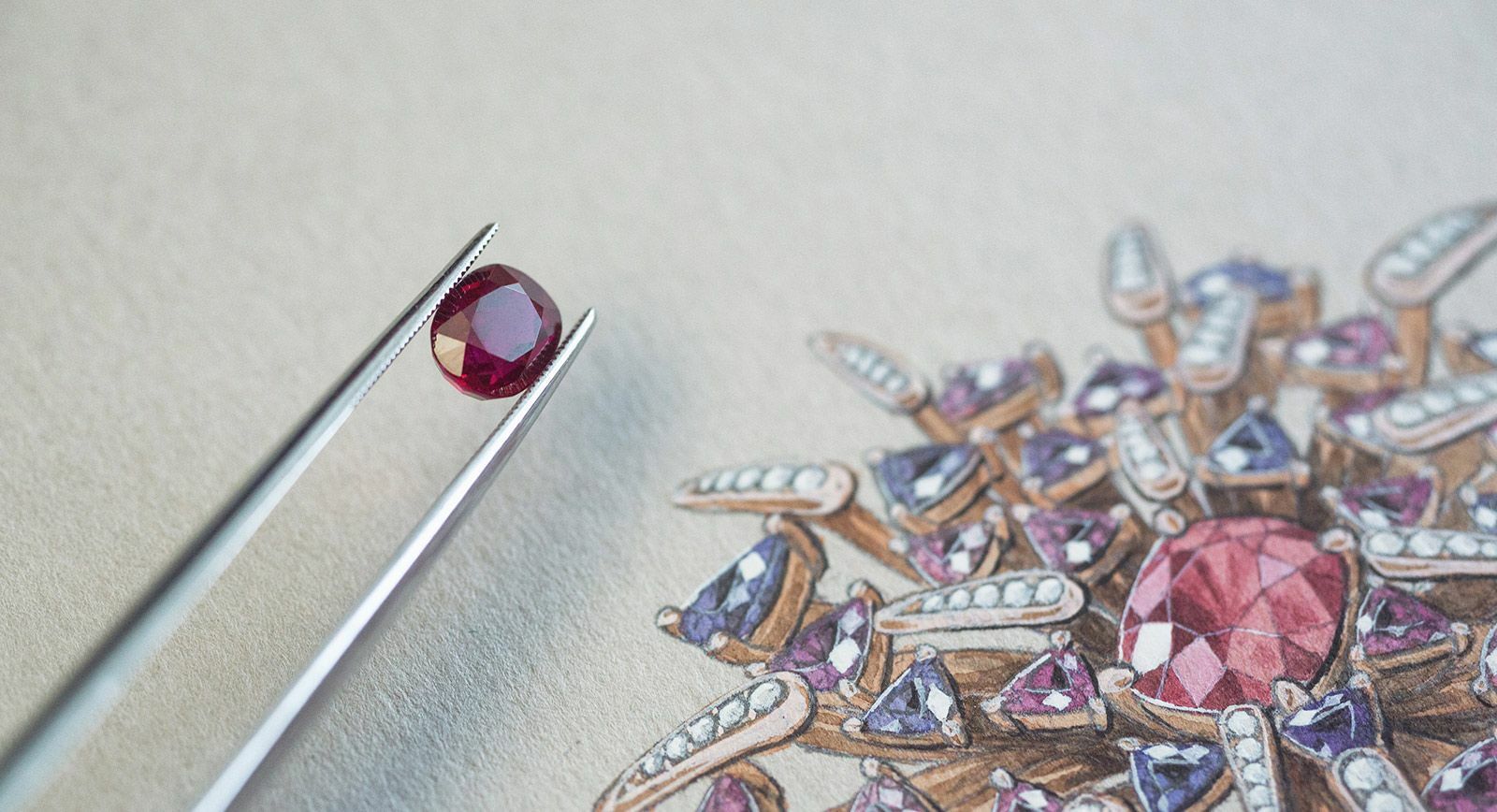The detailed image captures an exquisite close-up of a deep red or magenta ruby, securely held by a pair of silver metal tweezers, which enter the frame from the bottom left and grip the gem around the middle left. The clarity of the shot highlights the gleaming facets of the ruby, set against a white background. To the right of the ruby, there is a detailed jewelry design sketched on paper, featuring various gemstones in different shapes—triangles, cushions, and leaf-like patterns. The central piece of the design is another ruby, surrounded by blue and purple stones, along with small diamonds, collectively forming an intricate and radiant piece of jewelry. The bright lighting and high image quality make the details of both the ruby and the design clear and vivid.